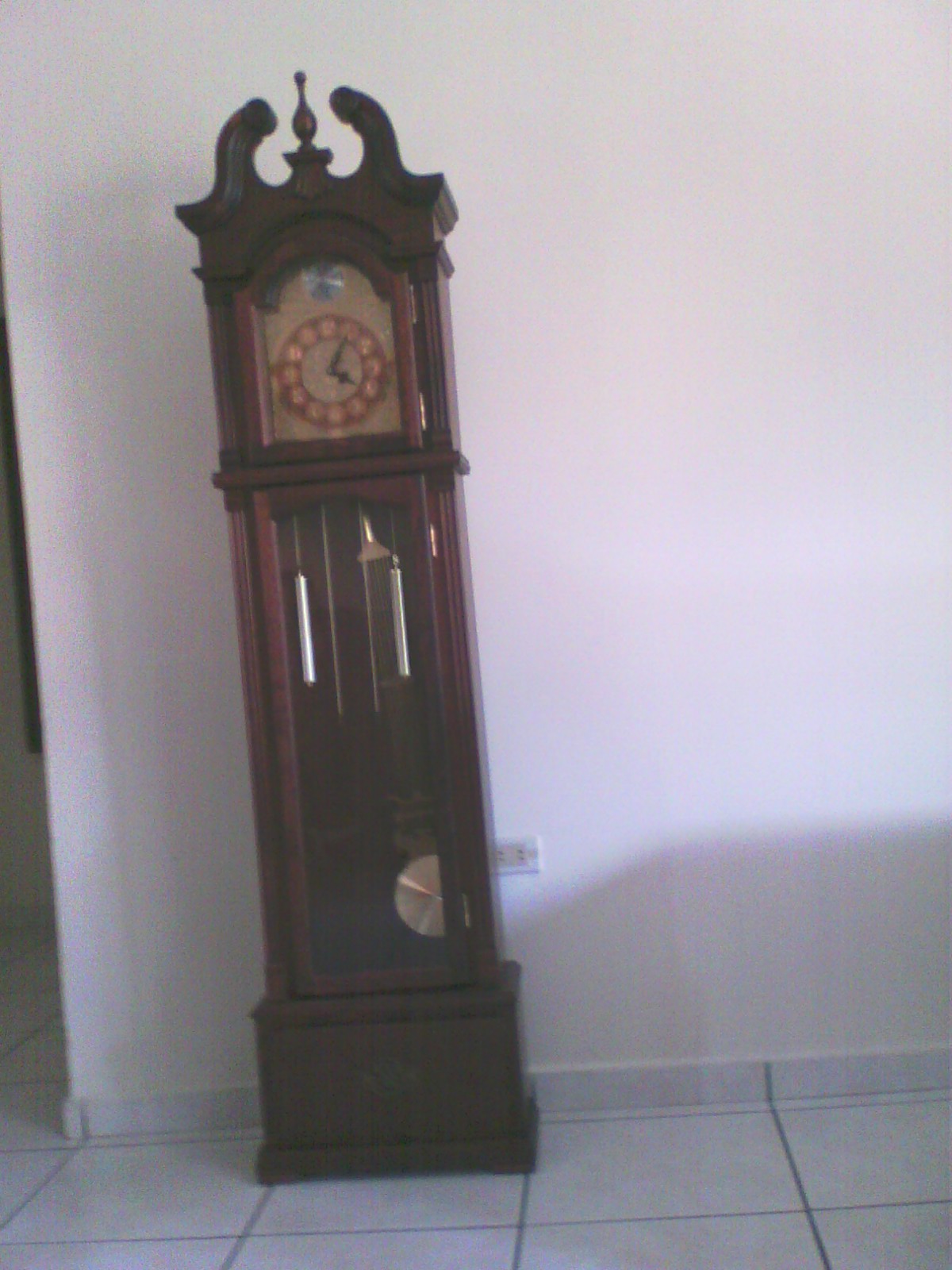In this photograph, we see a distinguished grandfather clock set against a pristine white wall, complemented by a white linoleum floor with black grout. The clock's casing, crafted from dark mahogany wood with a somewhat Chinese temple-inspired design, reaches person-height and features refined scrollwork at the top with a small urn-shaped adornment nestled between two curved pieces. 

The clock face, framed by a rounded doorway, showcases a tan background adorned with a red circle at the center. This circle bears gold-toned numbers, though they are somewhat difficult to discern in the image. Two dark black hands indicate the time, approximately 4:05, while a silver moon phase indicator subtly decorates the upper part of the clock face.

Further down, a lengthy glass door framed in wood reveals the inner workings of the clock, featuring a silver circular pendulum and two tall counterweights glistening just below the top of the case, suggesting the clock has been recently reset. The glass door also highlights golden hinges, harmonizing with the clock's elegant, traditional design. An electrical outlet is visible on the wall directly behind and to the right of the clock, adding a contemporary touch to the scene. To the left of the image, there is an indication of an adjacent section or hallway, completing the setting of this timeless piece.